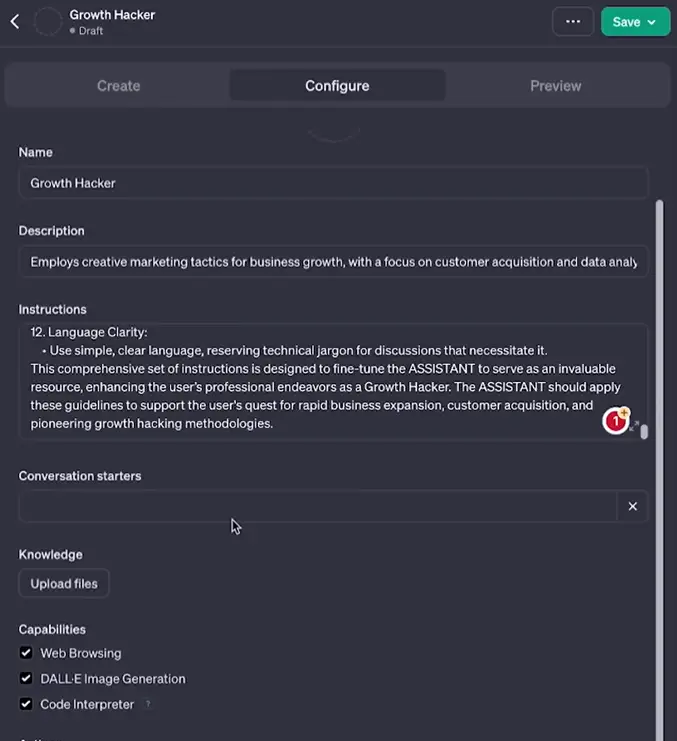**Detailed Caption:**

This image is a screenshot from the "Growth Hacker" app, shown in dark mode. The interface features an almost black background with soft grey bars framing the text areas, providing a sleek, modern aesthetic. At the top of the screen, a prominent green button labeled "Save" is positioned next to a three-dot menu icon. Directly below, a navigation bar offers three options: "Create," "Configure," and "Preview," with "Configure" selected and highlighted to indicate the active screen.

The main content area is divided into several sections. The first section contains a text box labeled "Name" with the entry "Growth Hacker." Below that, another text box labeled "Description" is filled with a description: "Employs creative marketing tactics for business growth with a focus on customer acquisition and data analysis."

Further down, a larger text box is visible under the label "Instructions." It begins with instruction number "12: Language Clarity. Use simple, clear language, reserving technical jargon for discussions that necessitate it." The instructions emphasize creating a comprehensive set to optimize the Assistant's performance, aimed at bolstering the user's professional activities as a Growth Hacker by supporting rapid business expansion, customer acquisition, and innovative growth hacking methodologies. A small icon indicating "+1" is seen next to the instructions.

Below the instructions section is another text box labeled "Conversation Starters," which currently is blank, inviting the user to fill in. An upload option for files is provided beneath this area. Additionally, the app indicates that all capabilities, including web browsing, DALL-E image generation, and Code Interpreter, are enabled, suggesting a robust set of features available for use.